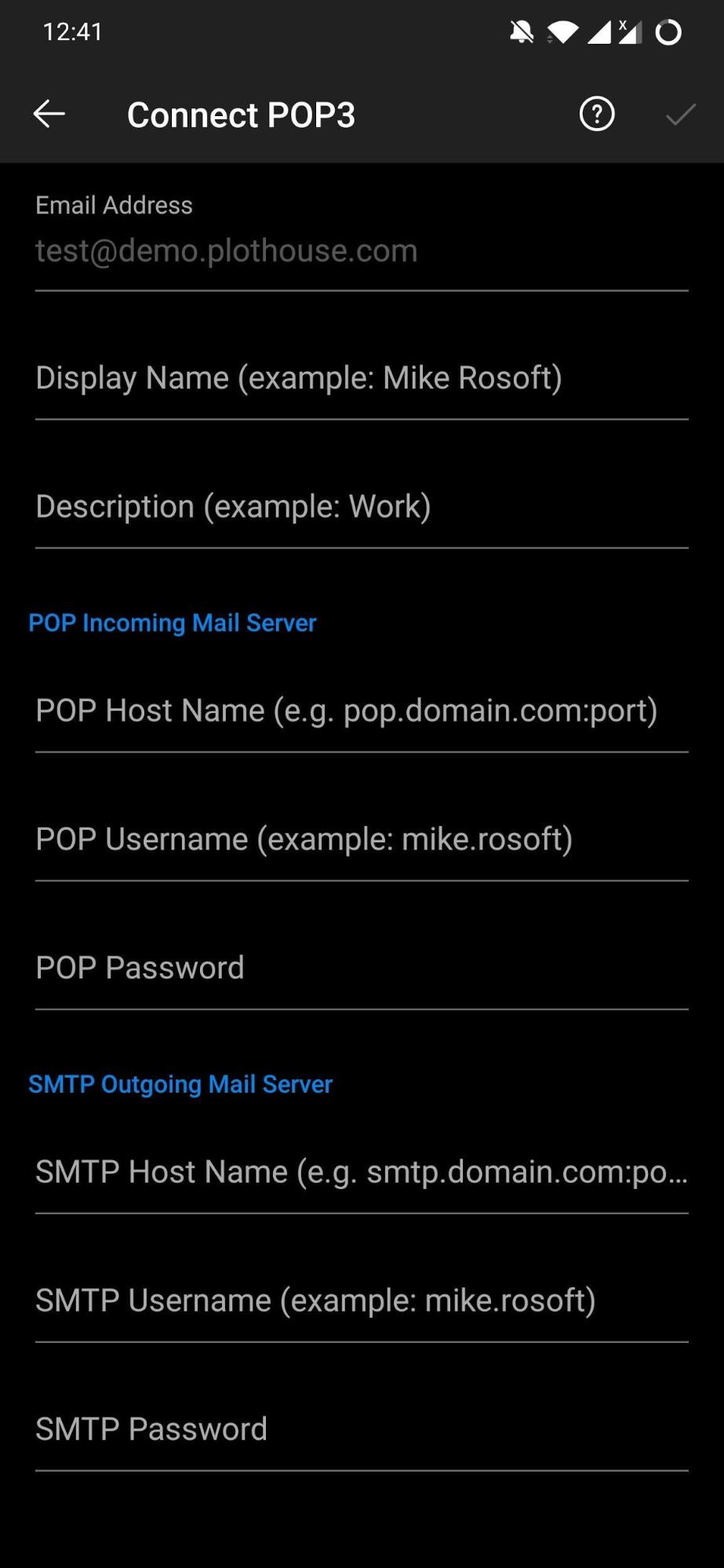This image depicts a settings section of a mobile device, featuring a configuration interface for email account setup. At the top of the image, there is a light gray navigation bar contrasting against the otherwise black background. On the left side of this gray bar is a white back arrow, and next to it, text that reads "Connect POP3." To the right, there is a help button represented by a white question mark inside a white circle, along with a checkmark.

Below the navigation bar, the black background hosts a vertical list of settings fields. The first entry is "Email Address," with an input bar beneath it for users to enter their email address. Following this is "Display Name," where an example name, "Mike Rosoft," is shown. The next field is "Description," here illustrated with the example text "example work."

Further down, the configuration details for the "POP Incoming Mail Server" are provided, including labels for "POP Host Name" with an example format (e.g., "pop.domain.com:port"), "POP Username" exemplified by "Mike.Rosoft," and "POP Password."

The list continues with settings for the "SMTP Outgoing Mail Server," including areas for "SMTP Host Name," "SMTP Username," and "SMTP Password." Notably, the actual credentials and hostnames are placeholders, intended to be customized by the user.

Overall, the image thoroughly delineates the fields necessary for setting up a POP3 email account on a mobile device, complete with example inputs for better guidance.